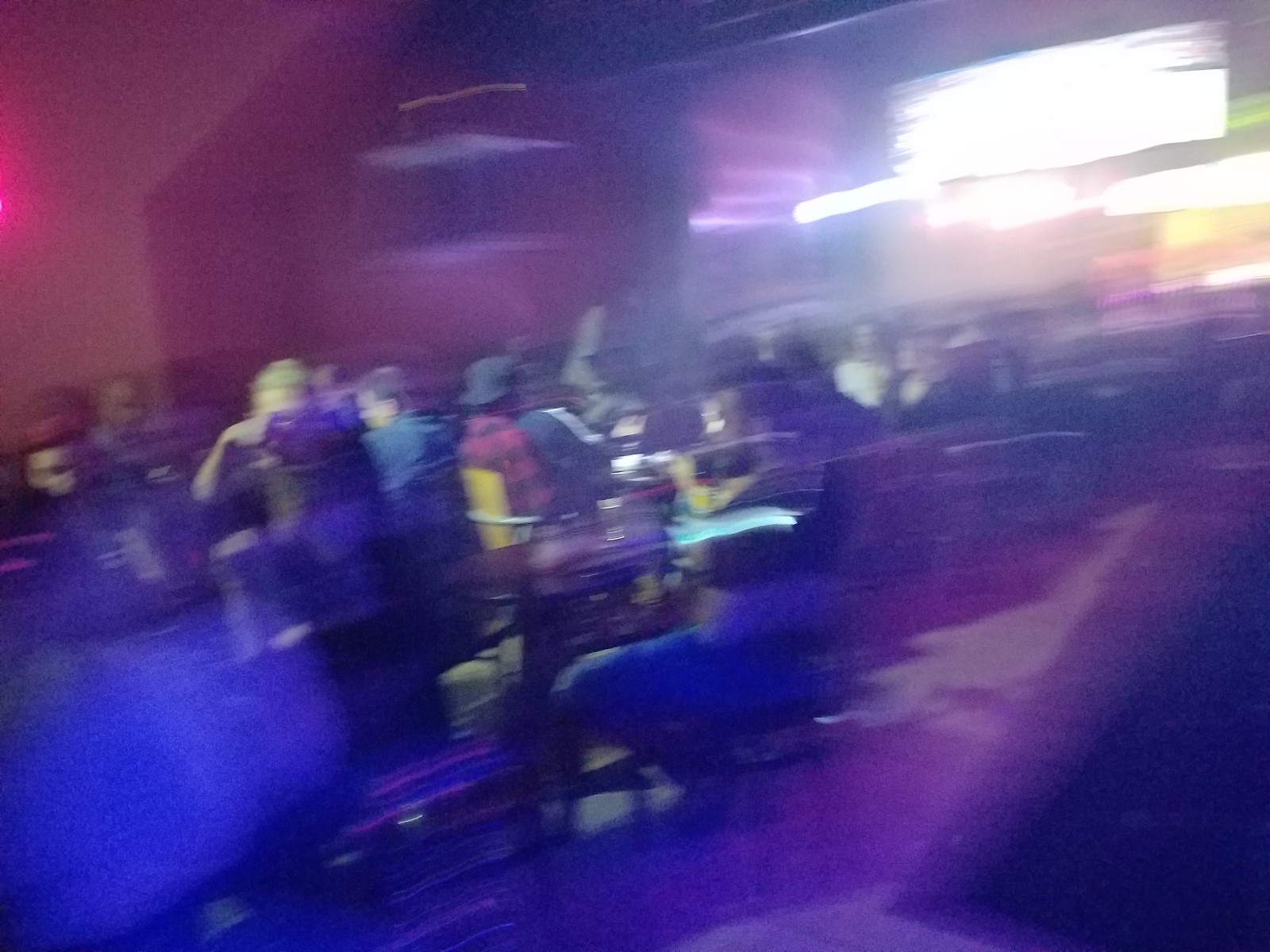This image captures a lively scene in what appears to be a restaurant. The overall color palette is dominated by purplish-red tones, giving the photo a warm and vibrant atmosphere. In the center of the frame, a group of people are gathered, some standing and others seated on high chairs around tall tables. A large panel of bright lights, potentially a TV screen, is visible in the background, adding to the dynamic ambiance. Above, several light fixtures hang from the ceiling, though they are slightly blurred in the photo.

To the left, a pink glow subtly illuminates part of the scene, enhancing the colorful setting. Among the individuals in the image, one man stands out in a red checkered shirt, while another can be seen wearing a blue shirt. Despite the slight blur, the photo effectively conveys a bustling and vibrant environment, likely capturing a moment of social interaction and enjoyment.